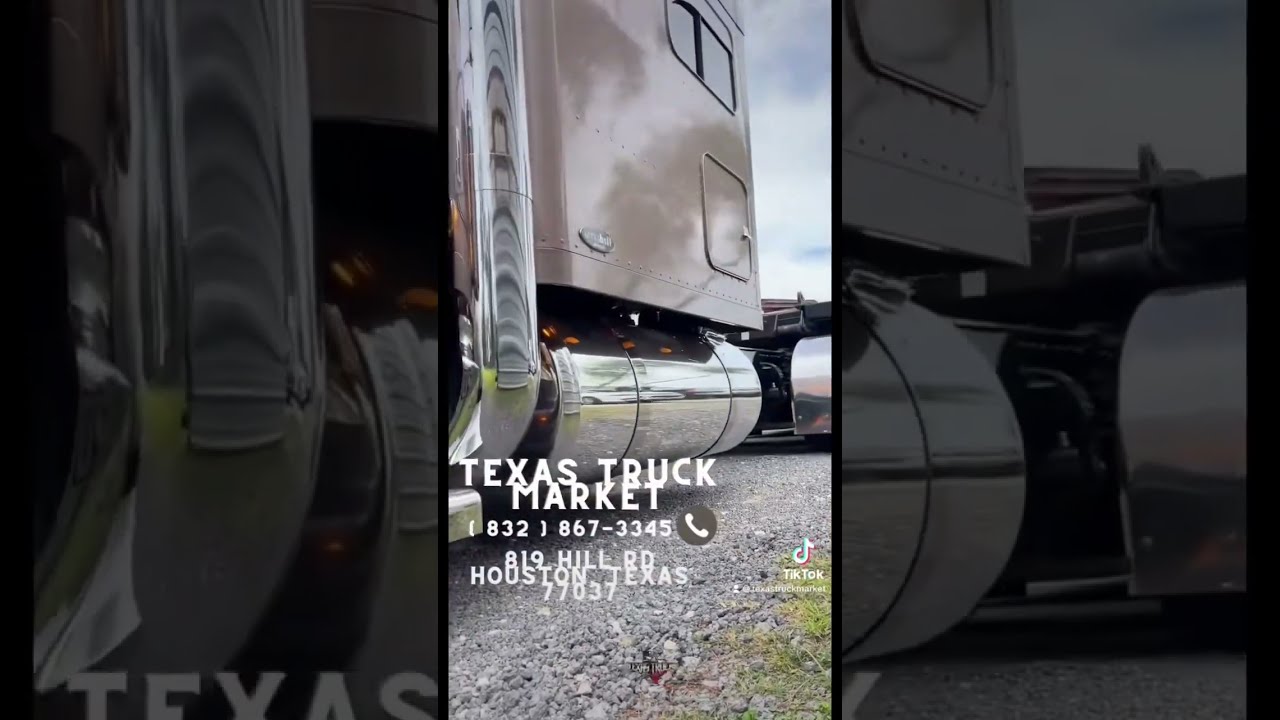The image is a close-up of a semi-truck's cab, highlighting its various features and advertisements for the Texas Truck Market. The truck is parked on a concrete surface with some visible grass to the right. The focus is on the middle third section of the truck, particularly on the shiny silver gas tank and the vertical metallic exhaust pipe that stands out prominently. The cab itself has a light bronze, almost taupe coloration, with a copper tone towards the top.

Above the gas tank, the truck's main body features a white and brown wall with a dark brown half-arch shape. There are two windows on the top right: the left one is curved like a half-circle, while the right one is rectangular. Additionally, there's a small door with a latch, possibly for adding gas. The shiny surfaces of the truck reflect surrounding objects, including a white truck.

In the center of the image, the text "Texas Truck Market" is clearly visible, written in white letters. Below this, the company’s contact information is provided: phone number 832-867-3345, and address 819 Hill Road, Houston, Texas, 77037. There's also a phone icon next to the phone number and a TikTok emblem in the right corner, suggesting multimedia engagement options. The overall impression is of a polished, well-maintained vehicle that serves as an advertisement for the trucking company’s services.